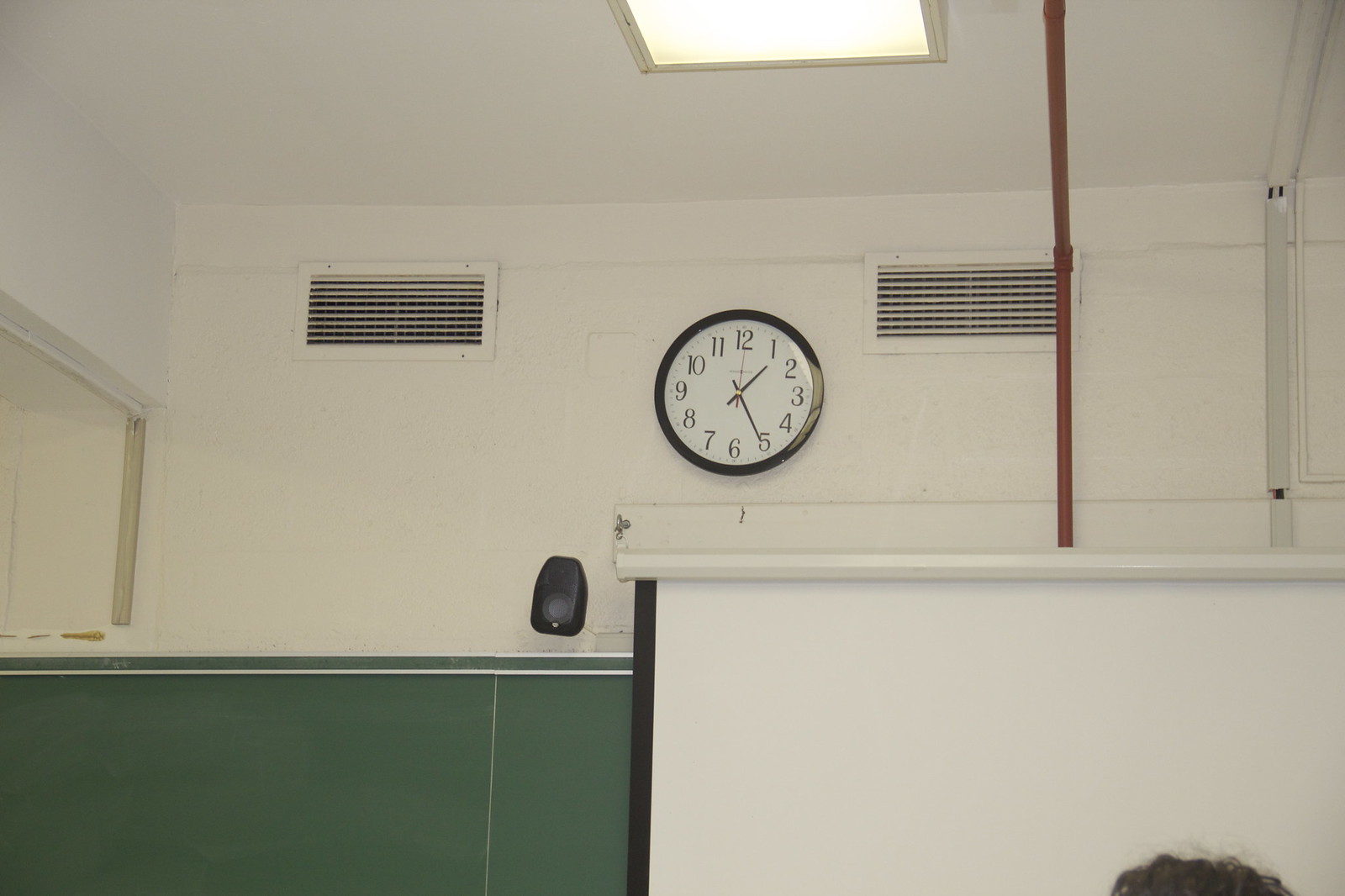The image shows the corner of a room, possibly an office or classroom. Visible on the wall are a white-faced clock with a black frame and Arabic numerals, which is flanked by two air conditioning vents. The clock has a long hand pointing at the 5 and a shorter hand between the 1 and 2. Above the clock, there is a black intercom unit. The walls, where some cubicles may be partially visible, feature contrasting sections: a white upper part and a green lower part. A red pole descends from the ceiling to a white ledge. Overhead, there is a square ceiling light and some visible pipes. To the right, there seems to be a whiteboard or chalkboard area, and a white doorway is partially visible. In the lower right corner of the image, the top of a person's head with dark hair is faintly visible in the foreground.